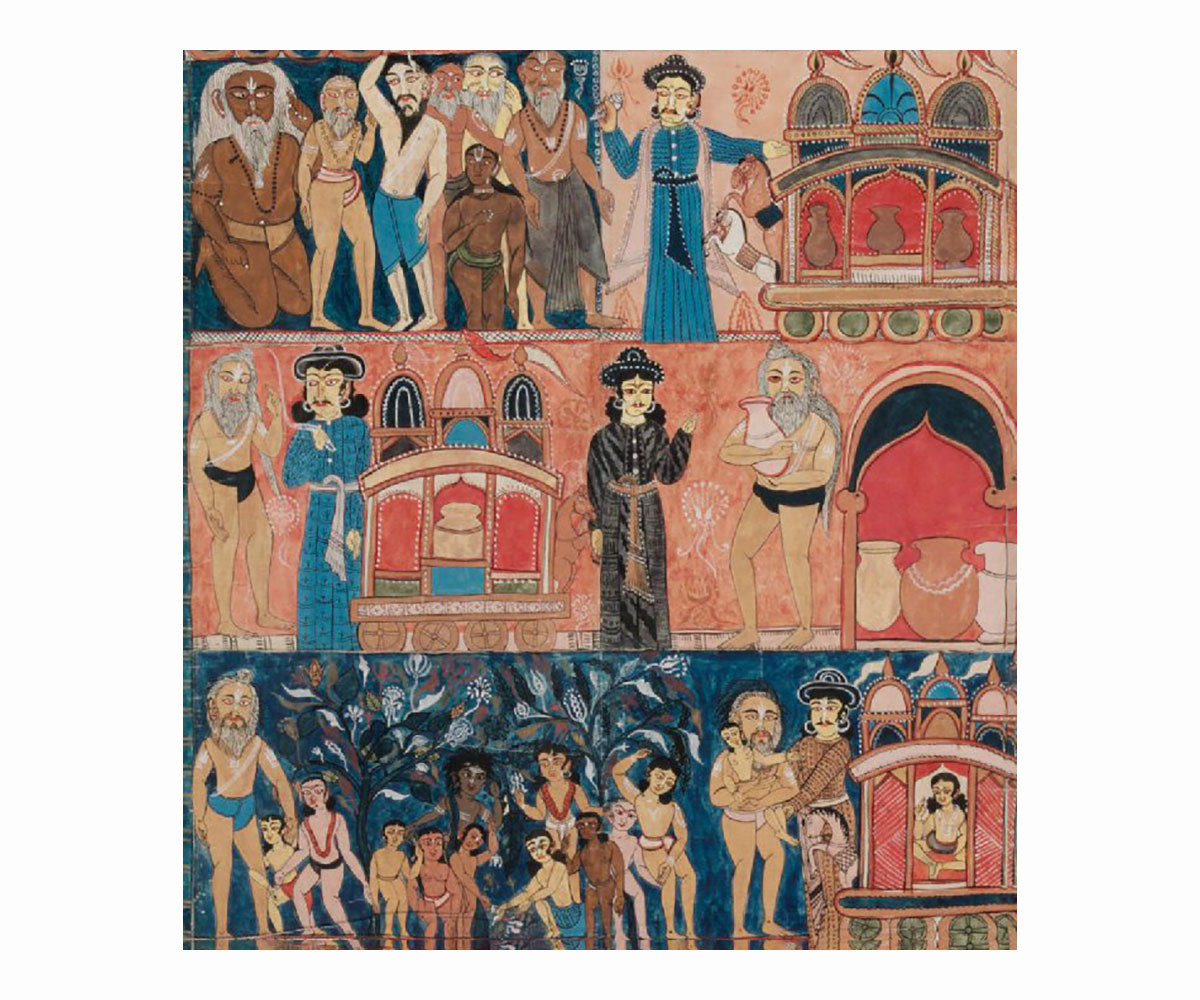This detailed painting, likely from an earlier time period, captures a vivid and colorful scene in a cartoony style, possibly of Asian descent. The artwork is divided into three horizontal panels, each depicting different scenarios.

In the top panel, an illustrious figure, perhaps Emperor Liang Kai, stands prominently to the right, garbed in a black hat and a long teal gown. Surrounding him are eight other figures, dressed in simpler clothing, some in loincloths and others in long, flowing garments. They appear to be inspecting a horse-drawn cart laden with various goods, including vases and perhaps rocking horses.

The middle panel also features Emperor Liang Kai and introduces a woman dressed in a black gown and hat, who could be of significant status. They are flanked by two servants offering water from pitchers. The ambiance here suggests a market or a courtyard scene, where goods are being shown or traded.

The bottom panel is the most populated, showcasing around fifteen people and a small child. One central figure is inside a structure resembling a castle, while the others, clad in minimal clothing or servant attire, gather outside. Among them is a man holding a smaller woman in his arms, hinting at a sale or trade, adding a layer of complexity and potential drama to the narrative depicted in this vibrant and dynamic painting.